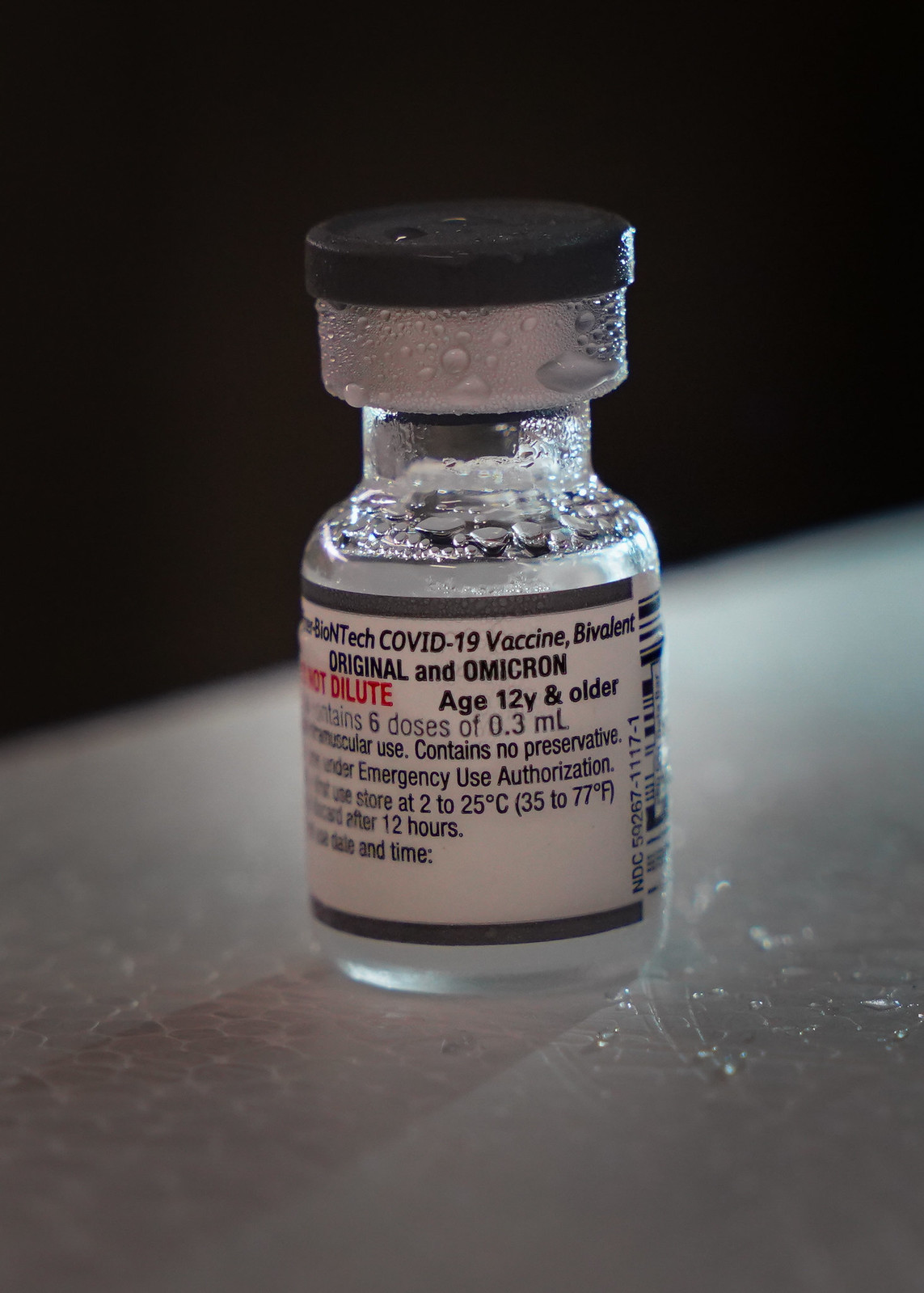This image features an unopened vial of the Pfizer-BioNTech COVID-19 mRNA bivalent vaccine, designed for both the original strain and the Omicron variant. The vial is positioned upright on a white surface against a dark background, with noticeable condensation droplets forming around it and pooling on the surface below. The vial has a distinctive black lid and a silver band around its neck, and there's a clear, slightly teal-tinted glass body. The label, in Times New Roman font, indicates the vaccine is for ages 12 and older, contains six doses of 0.3 milliliters each, and specifies "Do not dilute" in red letters. Additional details include it containing no preservatives, being authorized for emergency use, and storage requirements of 2 to 25 degrees Celsius (35 to 77 degrees Fahrenheit). There's also a designated space on the label to note the date and time the vial was opened, with instructions to discard it after 12 hours. The overall presentation of the vial with its condensation and reflective surface gives it a slightly glowing appearance.